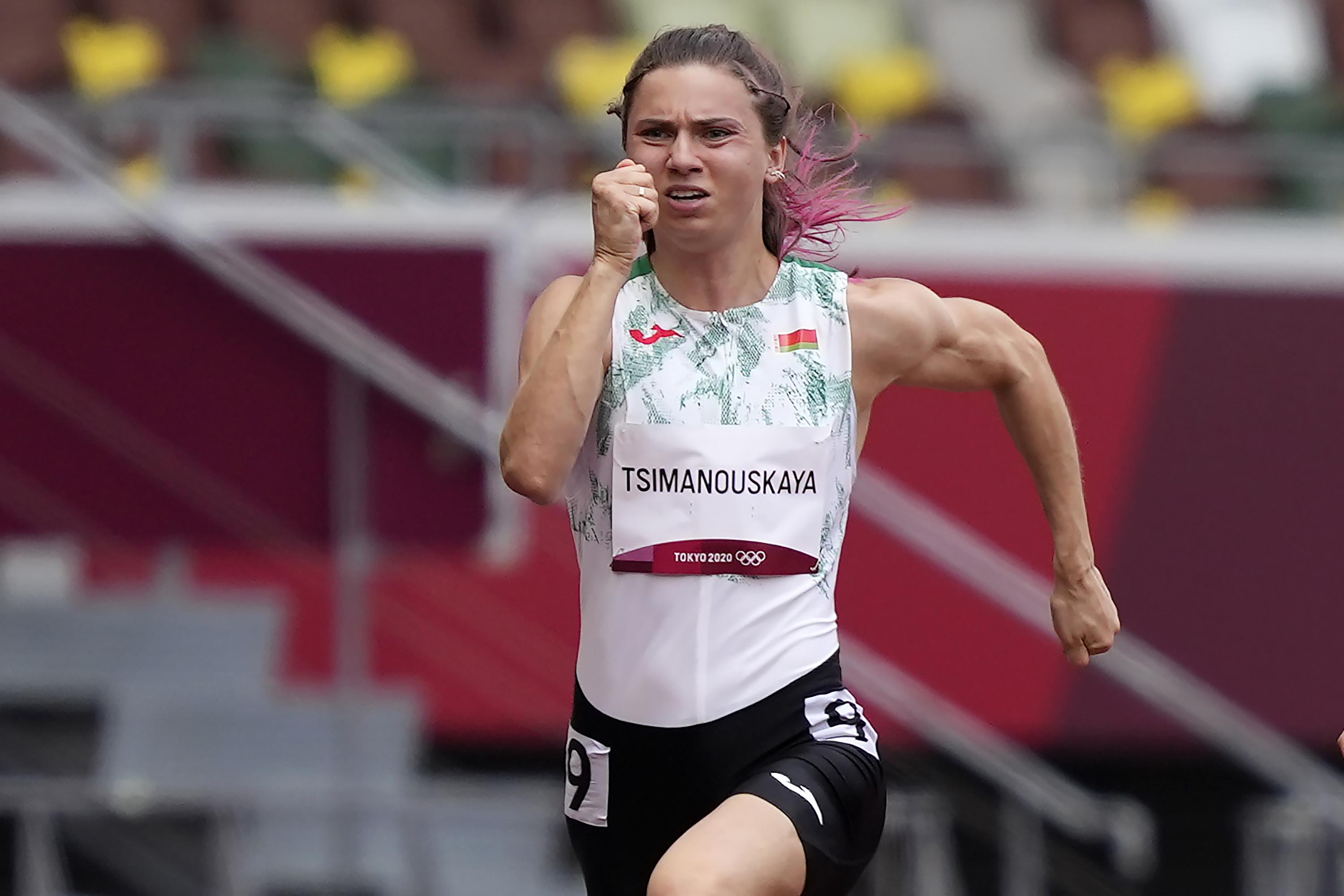This detailed image captures a determined female marathon runner, likely participating in the Tokyo 2020 Olympics. The photo, taken in landscape orientation, focuses on the athlete from the top of her head to about mid-thigh, centered within the frame as she runs toward the left side. She has dark brown hair pulled back into a ponytail with distinctive pink highlights. Her facial expression is intense, displaying hard breathing and eyes slightly narrowed, reflecting the effort and pain of the race.

She wears a white cut-off sleeve jersey adorned with light green patterns, featuring a red and light yellow flag, and a curving red design near the collar. Attached to her chest is a white placard that reads "T-S-I-M-A-N-O-U-S-K-A-Y-A" above an arc-shaped burgundy area that says "Tokyo 2020" accompanied by the Olympic rings in white. Her black running shorts also feature the number "9" in black on the sides with a small white label behind the number.

Her athletic physique is evident, with muscular arms and a visible vein in her bicep. Her left arm is extended behind her back, while her right hand is raised near her face, both captured in dynamic running motion. The background reveals a blurred crowd of spectators seated on red concrete steps with a guardrail above them, emphasizing the runner as the focal point of the image.